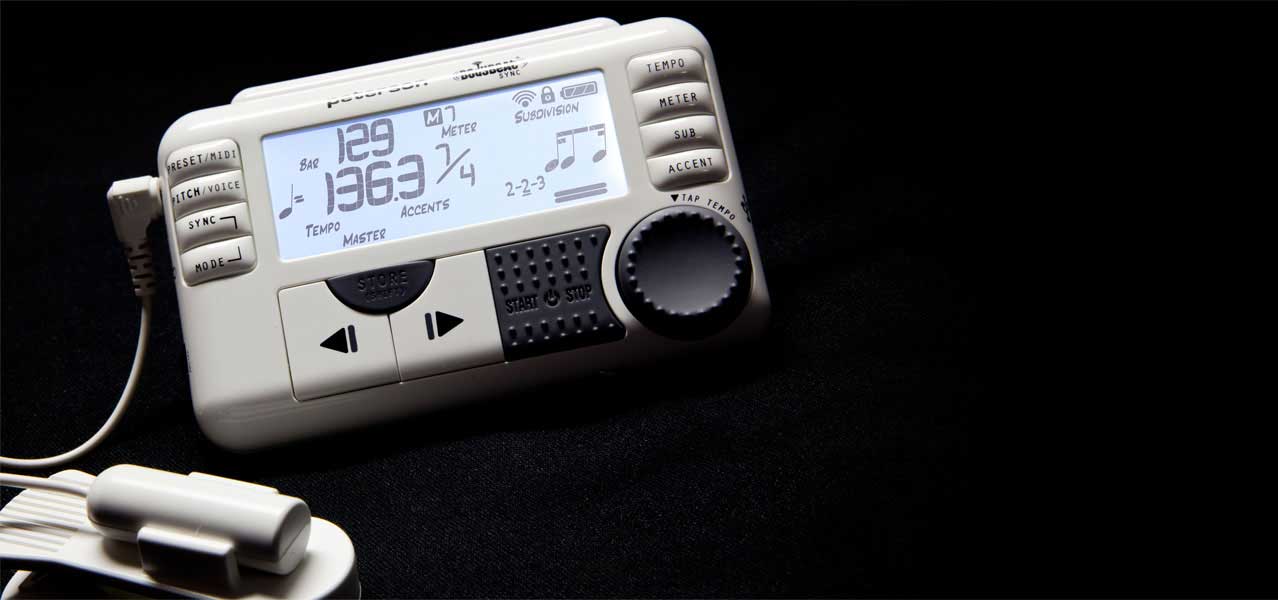The image depicts a white, rectangular metronome with rounded corners set against a completely black background, drawing all attention to the device. It features a digital screen displaying various numbers such as 129 and 136.3, along with terms like "tempo," "accents," and "master." Musical symbols are visible on the right side of the screen. The left side of the metronome is equipped with buttons labeled "preset/midi," "pitch/voice," "sync," and "mode," while the right side has buttons for "tempo," "meter," "sub," and "accent," as well as start/stop controls and fast forward or go backward functions. A black circular dial is located at the bottom right-hand corner. A wire is plugged into the side of the metronome, likely connecting to headphones or another instrument. The lighting focuses solely on this device, highlighting its details and functionality in a clear and well-lit setting.